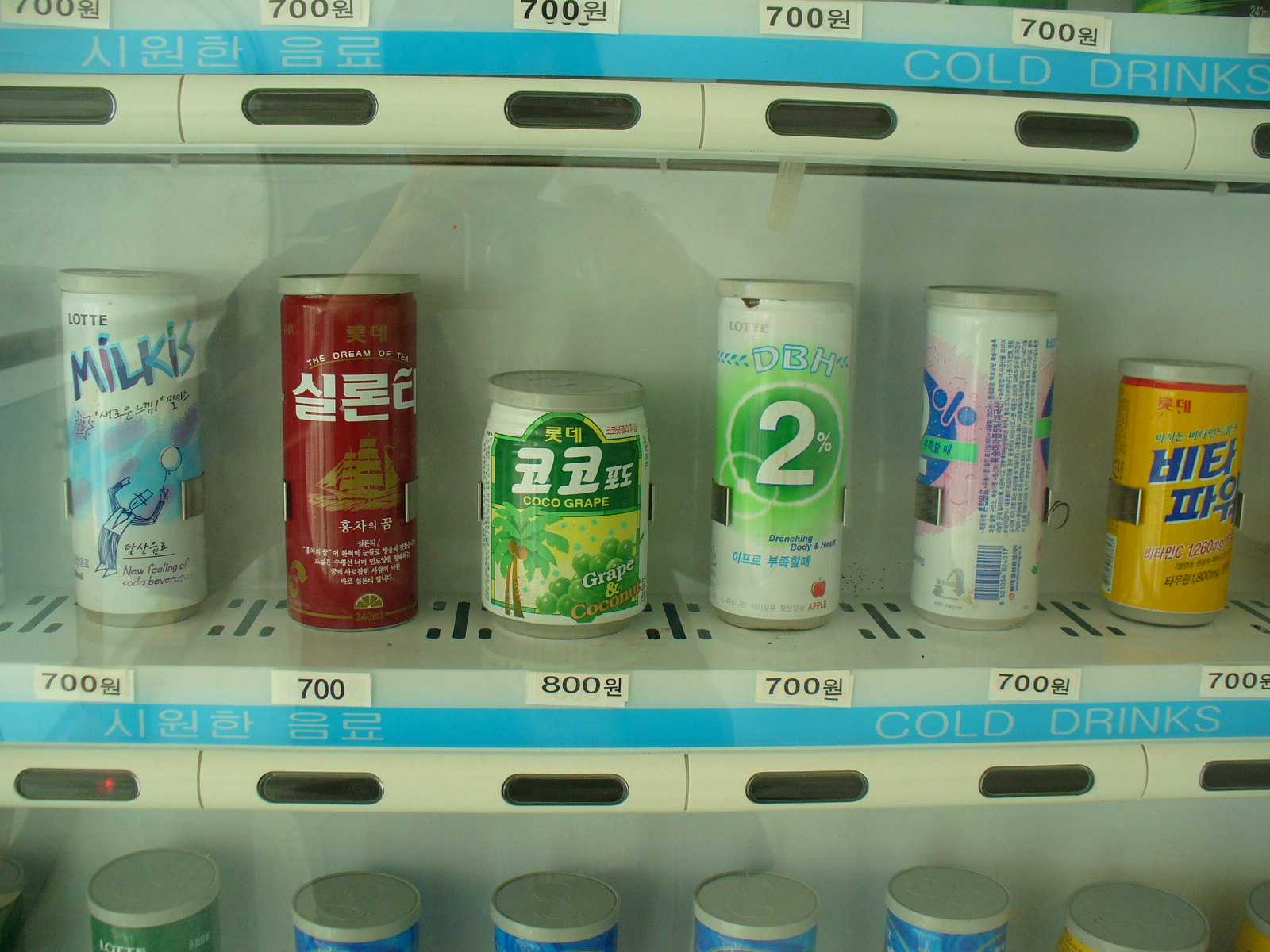The image depicts a close-up of a Japanese vending machine showcasing six different cold drinks. The drinks, all in cans, are arranged on a metal shelf behind a glass front. Each can is distinctly colored: the first is white, the second red, the third green, the fourth white with green accents, the fifth pink and white, and the sixth a shorter yellow can with blue writing. The price strip, which appears to be blue, displays prices in yen, specifically 700 yen for most cans and 800 yen for the smaller ones. Though the majority of text is in Japanese, the words "cold drinks" are prominently displayed in English. The overall scene features a variety of colors including gray, green, light blue, black, dark blue, red, maroon, gold, and yellow. There is some visible reflection on the glass, indicating that the photo was taken up close, likely from the perspective of a potential customer.